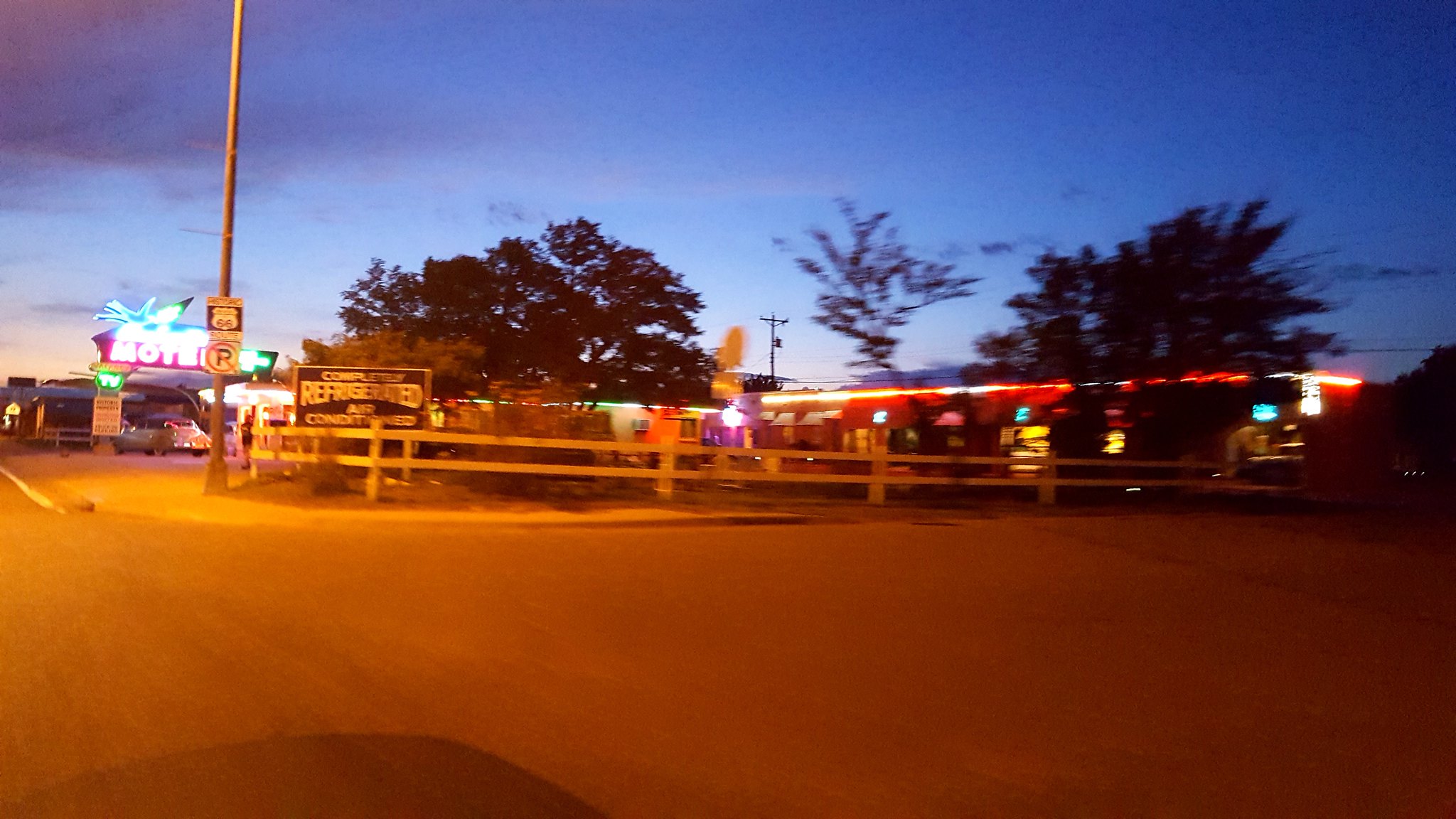The image captures a street corner at dusk, with a twilight blue sky that hints at the day's end. In the background stands a one-story motel adorned with vibrant, multicolored neon lights in reds, blues, and whites. The motel sign to the left features large, pink neon letters spelling “MOTEL,” though a utility pole obstructs the last letter. Above “MOTEL,” there is a blue neon design, and directly beneath the sign, an old-timey car is parked. The larger, rectangular wooden sign near the motel advertises that it’s fully refrigerated and air-conditioned. A white picket fence lines a central area in the photo, behind which you can spot trees turning into dark silhouettes against the encroaching night. The streetlights are on, reflecting off the road, and there’s a sign with a black "P" inside a red circle with a slash, indicating no parking. The hazy orange and white glow in the background suggests a gas station or filling station, its pumps illuminated in yellow. There's also a faint shadow of the vehicle from which the photo was taken, visible in the bottom left corner of the image.